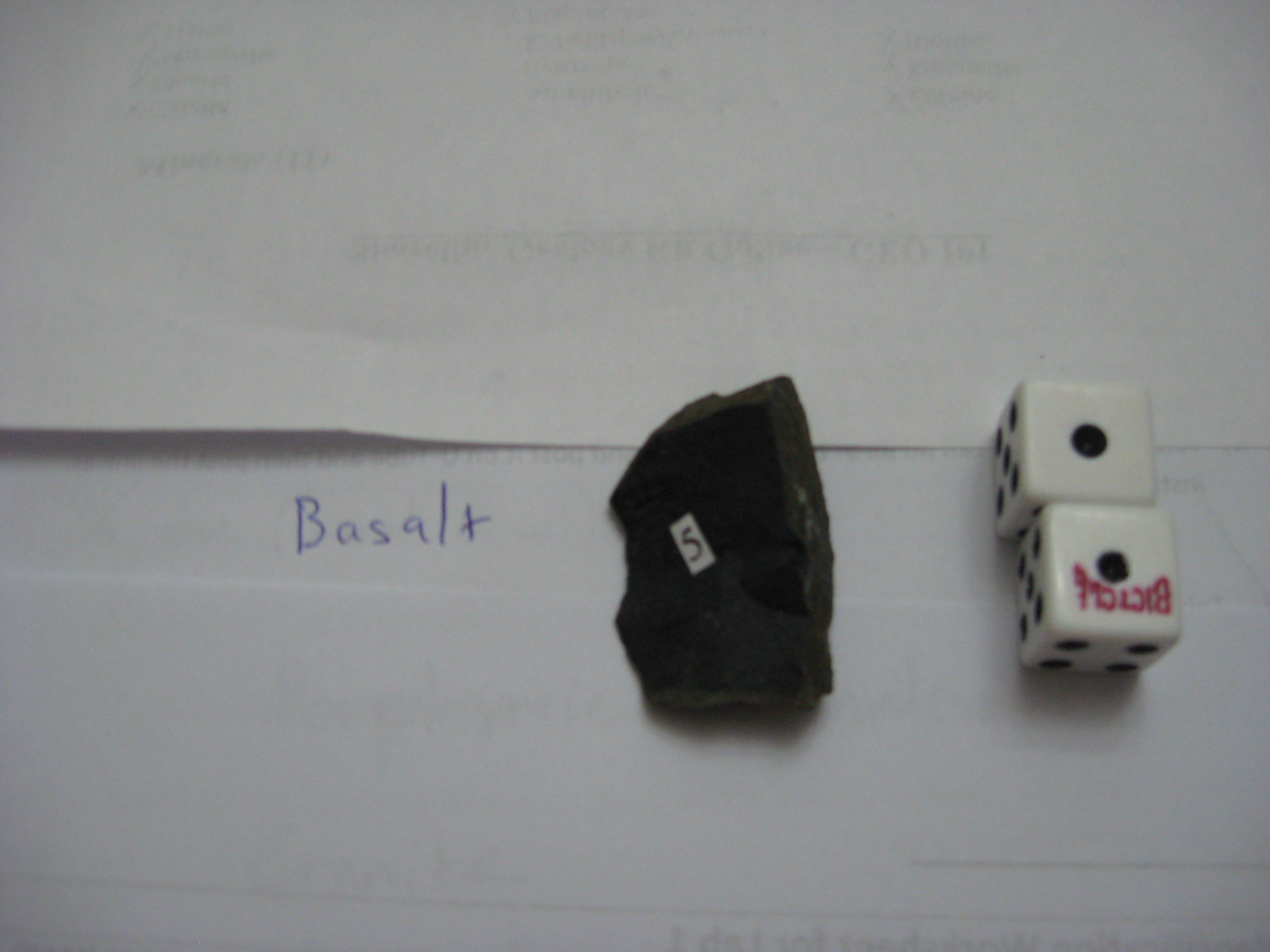The image features three overlapping pieces of paper in the background, with the two outer sheets positioned upside down, revealing blurred, unreadable text through the paper. Between these two sheets, the middle paper clearly displays the word "Basalt" written in blue ink. Centrally positioned on top of the papers is a black basalt rock, identifiable by a white sticker with the number 5 in black font affixed to it. To the right of the rock, two dice are stacked on top of each other with both showing the one dot facing up, indicating "snake eyes." The lower die appears to have the word "Bicycle" faintly visible in red letters, though slightly obscured.